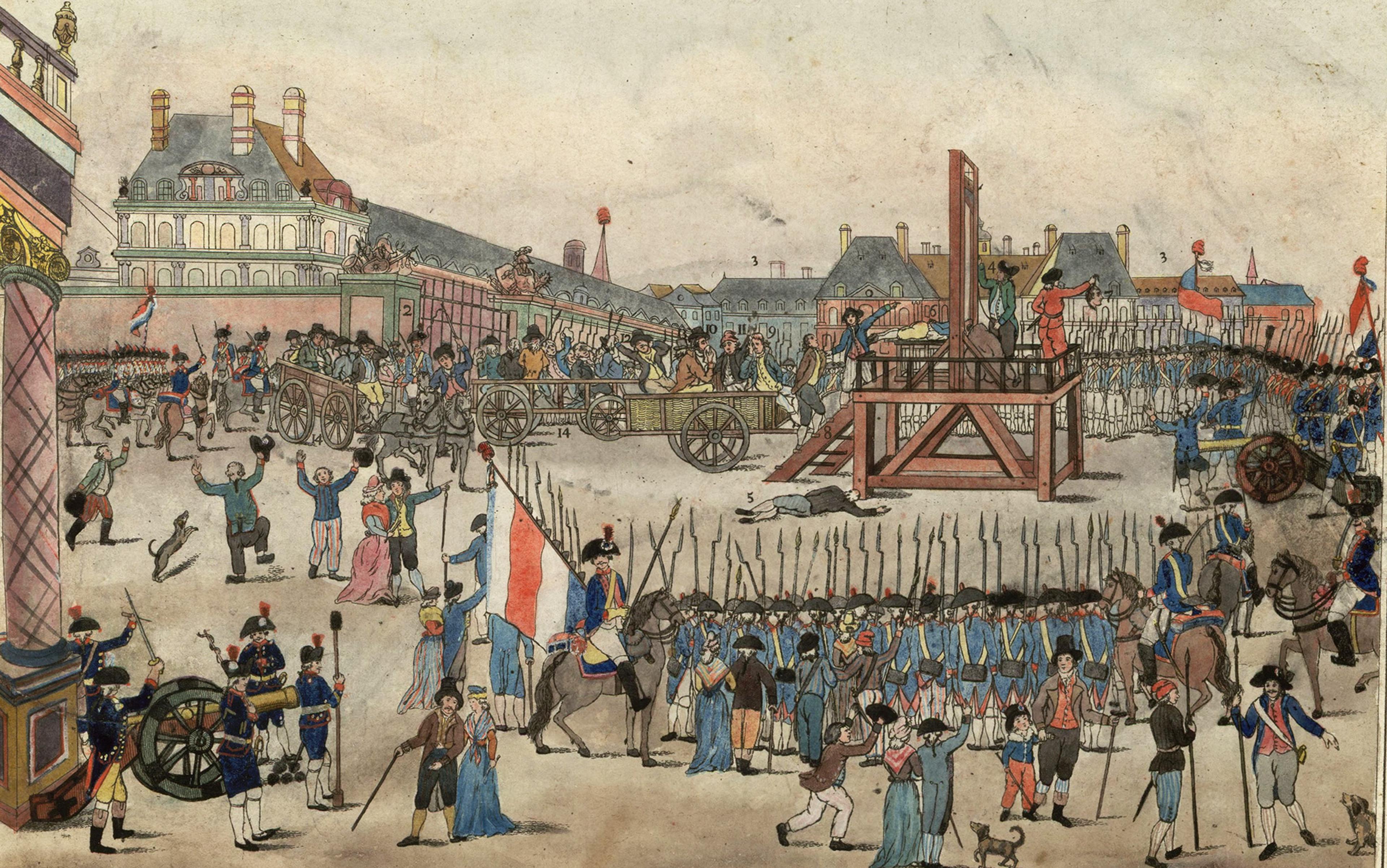This detailed and colored image, reminiscent of an old Civil War or World War I-era scene, appears to be an 1800s or possibly 1700s depiction of a public execution in France. The illustration showcases a bustling city square within the city walls, with a dramatic sky painted in white and light clouds. In the background, a row of connected buildings stands, featuring a prominent long structure with numerous windows and three visible chimneys, all roofed in shades of gray and brown.

Prominently, there’s a French flag with alternating stripes of white, red, and blue amidst a dense assembly of soldiers dressed in dark blue jackets, armed with muskets and bayonets. Horses and cannons are strategically positioned within the square. Amid the soldiers and onlookers, there's lively interaction including men and women walking with dogs, children, and people enthusiastically waving hats.

Central to this intense scene is a raised platform upon which a guillotine stands ominously. Two men atop are holding up a recently severed head, signaling the somber reality of an execution. The decapitated body lies at their feet, confirming the brutal nature of the event. Surrounding the execution site are wagons filled with people, likely witnessing the grim event, pulled by horses and facing an organized, disciplined line of soldiers.

This vivid and historically rich painting or drawing serves as a detailed snapshot of a dramatic public moment, rich with elements of military presence, public gathering, and execution, capturing a significant historical ambience through its intricate details and colored presentation.